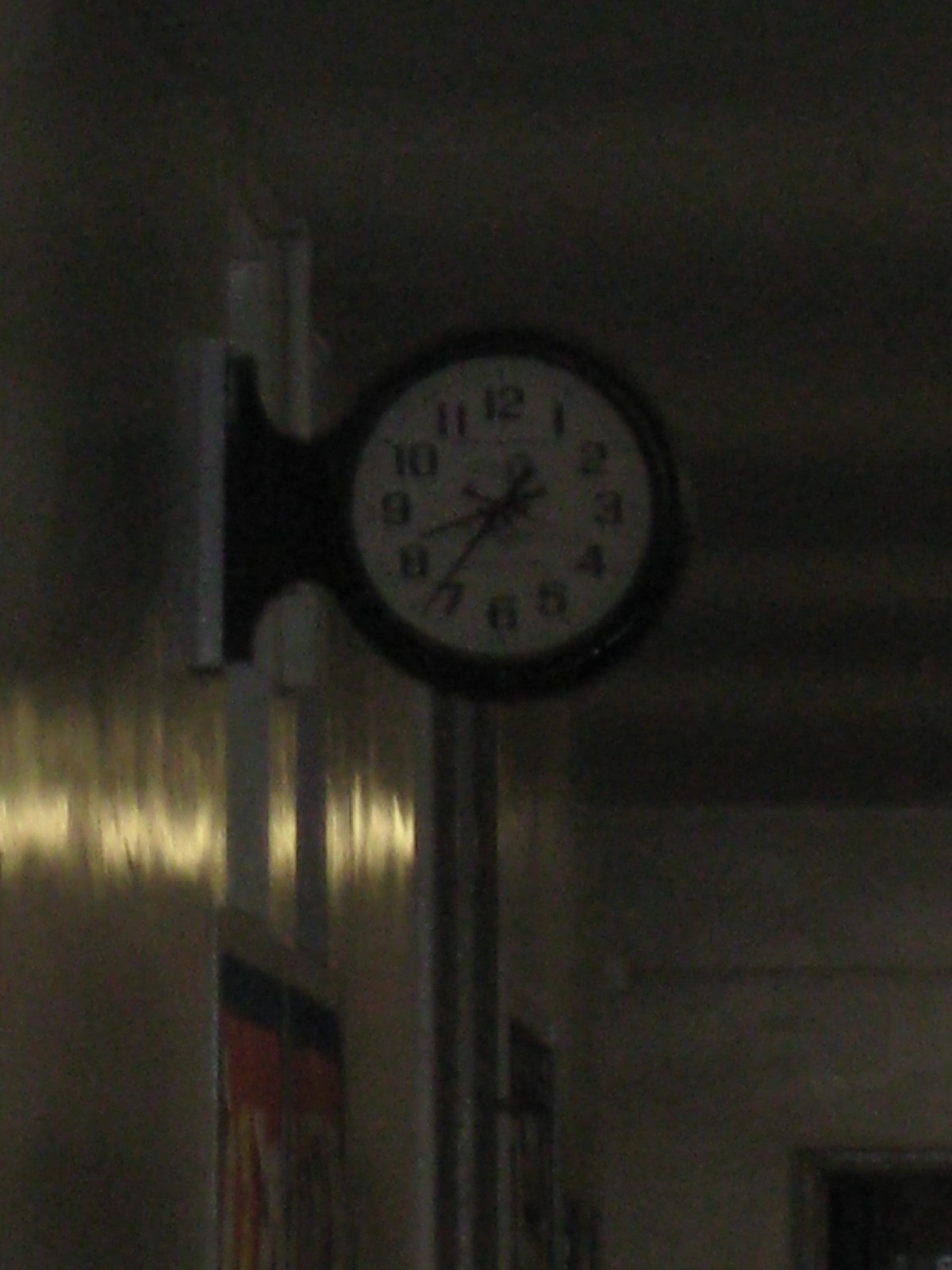The image features a clock mounted on a hallway wall, likely belonging to a building's interior passage. The hallway walls are finished in plaster and exhibit a shiny texture with a yellowish tint. In the background, a door frame is visible. The clock, designed to protrude from the wall near the ceiling, is mounted on a black bracket and encased in a black housing, allowing it to be visible from both directions. The clock face presents black numerals arranged clearly around its circumference, accompanied by hour, minute, and second hands, indicating a time of approximately 8:36. A reflection of light stretches across the wall, suggesting the presence of a row of small windows on the opposite side. Additionally, a few indistinct posters adorn the wall, with the closest poster displaying a mix of red, yellow, and dark colors.